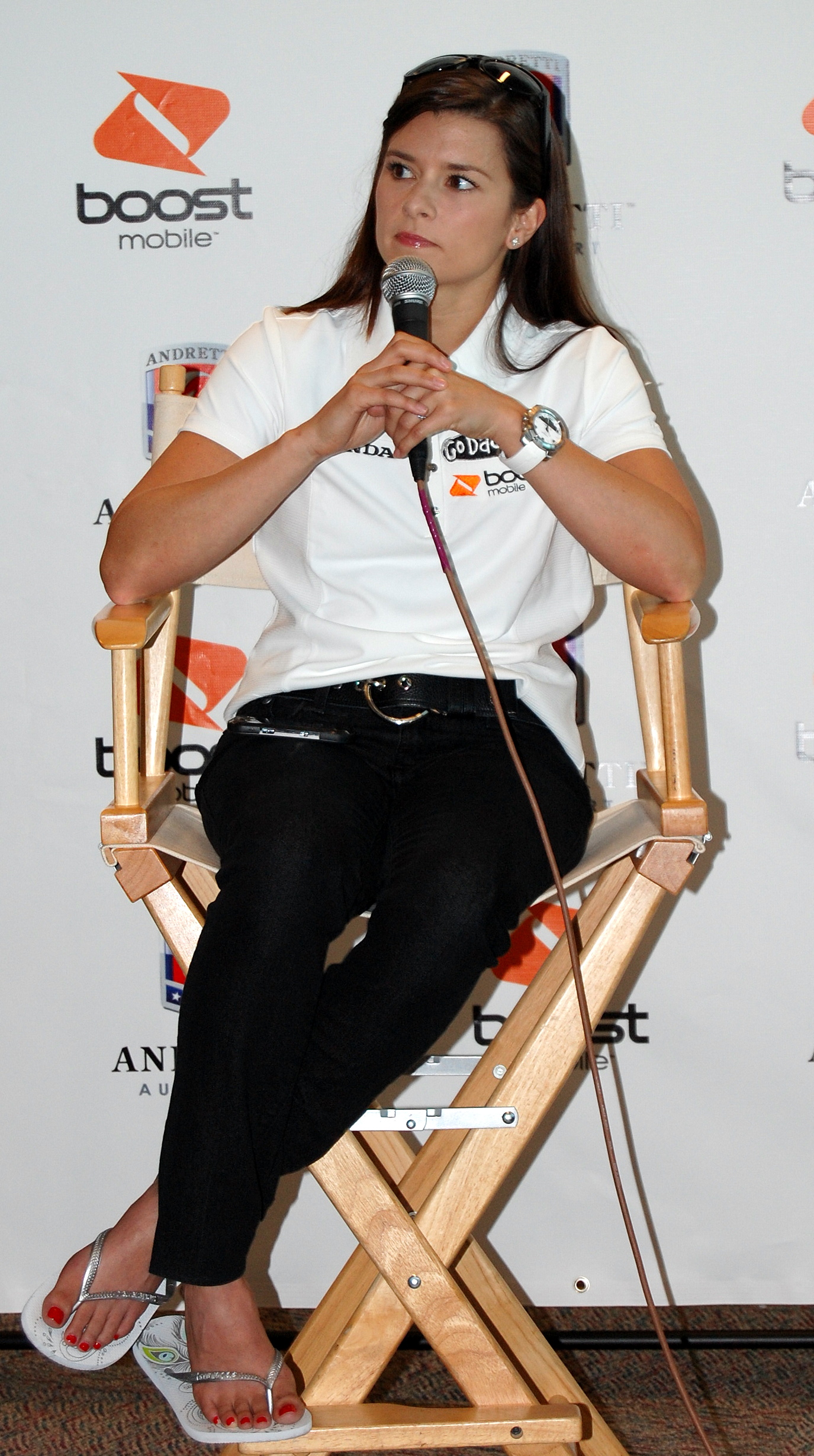The photograph captures a woman seated in a brown, high director's chair with wood and metal construction, featuring a cloth seat and back. She is wearing white sandals with silver tops, black pants secured with a black belt, and a white polo t-shirt. Adorning her feet are red toenail polish, and she sports small diamond stud earrings and a white watch. Her dark reddish-brown hair is accompanied by black sunglasses atop her head, and she wears pink lipstick.

In her hand, she holds a microphone with a visible cord extending from the bottom to the top. She has long dark hair, dark eyes, and sets of white pearl-looking earrings. Her attire includes a polo shirt emblazoned with a few logos, notably "Honda," "GoDaddy," and an orange "Boost Mobile" logo with black text, though part of the shirt is slightly obscured, possibly hiding more information.

Behind the woman, the backdrop is covered with a repeating pattern of logos, prominently featuring the "Boost Mobile" logo—orange triangle shapes with their bases facing each other and the text in black. One of the logos is obscured by her positioning. The scene gives the impression she is part of an event or interview, as she is looking slightly to the left, potentially attentive to someone speaking off-frame.

For additional context or further information visit www.FEMA.gov.